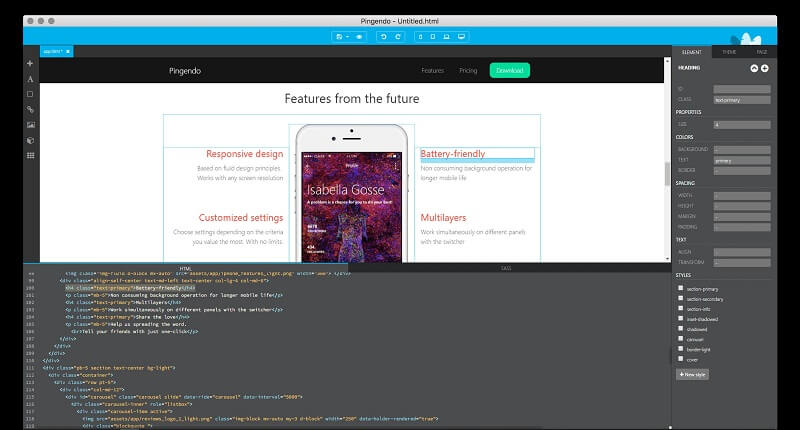A detailed screenshot of a website interface is displayed on a desktop or laptop screen. At the top, a gray bar labeled "Pengendo Untitled.html" is present, followed by a blue bar underneath. On the right side, a drop-down menu featuring various settings is visible, while the left side showcases additional settings icons. The bottom half of the screen reveals lines of computer code; the text is predominantly white with numerous gold characters and some blue elements, with gold being more prominent.

Centrally located on the page is a section with a white background, showcasing an image of an iPhone. The iPhone screen displays "Isabella Gauze," suggesting a music-related context. Below the iPhone image, key features are listed: "Responsive Design, Customized Settings, Multiplayers, Battery-Friendly, Features from the Future."